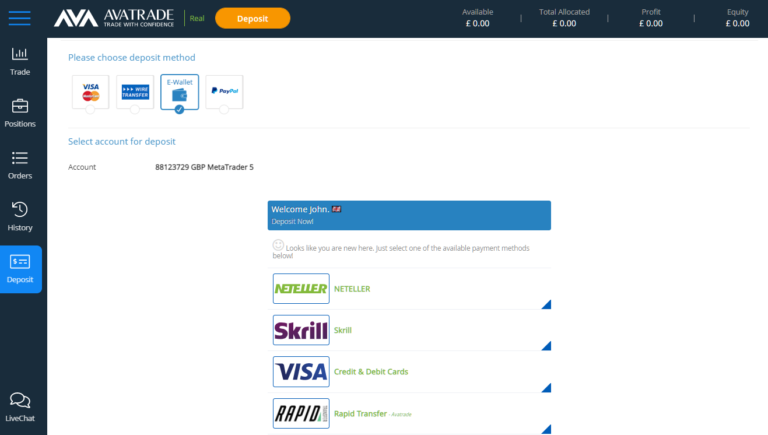This image is a screenshot from a page on the AvaTrade website. At the top of the page, the AvaTrade logo is prominently displayed along with a tagline "Trade with Confidence." Below this, an orange, rounded rectangle button labeled "Deposit" is visible.

The left sidebar features a vertical menu with the following labels: "Trade," "Positions," "Orders," "History," and "Deposit." At the top of the page, there are icons representing various deposit methods, including Visa, wire transfer, e-wallet, and PayPal. An account number and the heading "MetaTrader 5" are also displayed prominently.

In the center of the screen, there is a blue area welcoming the user with a message, "Welcome, John. Deposit now." Underneath this, there is a list of deposit options such as Neteller, Skrill, Visa, and Rapid, each with clickable sections.

At the top, several financial metrics are displayed with values in British Pounds (GBP): "Available: £0.00," "Total Allocated: £0.00," "Profit: £0.00," and "Equity: £0.00." These metrics are likely placeholders until transactions are made.